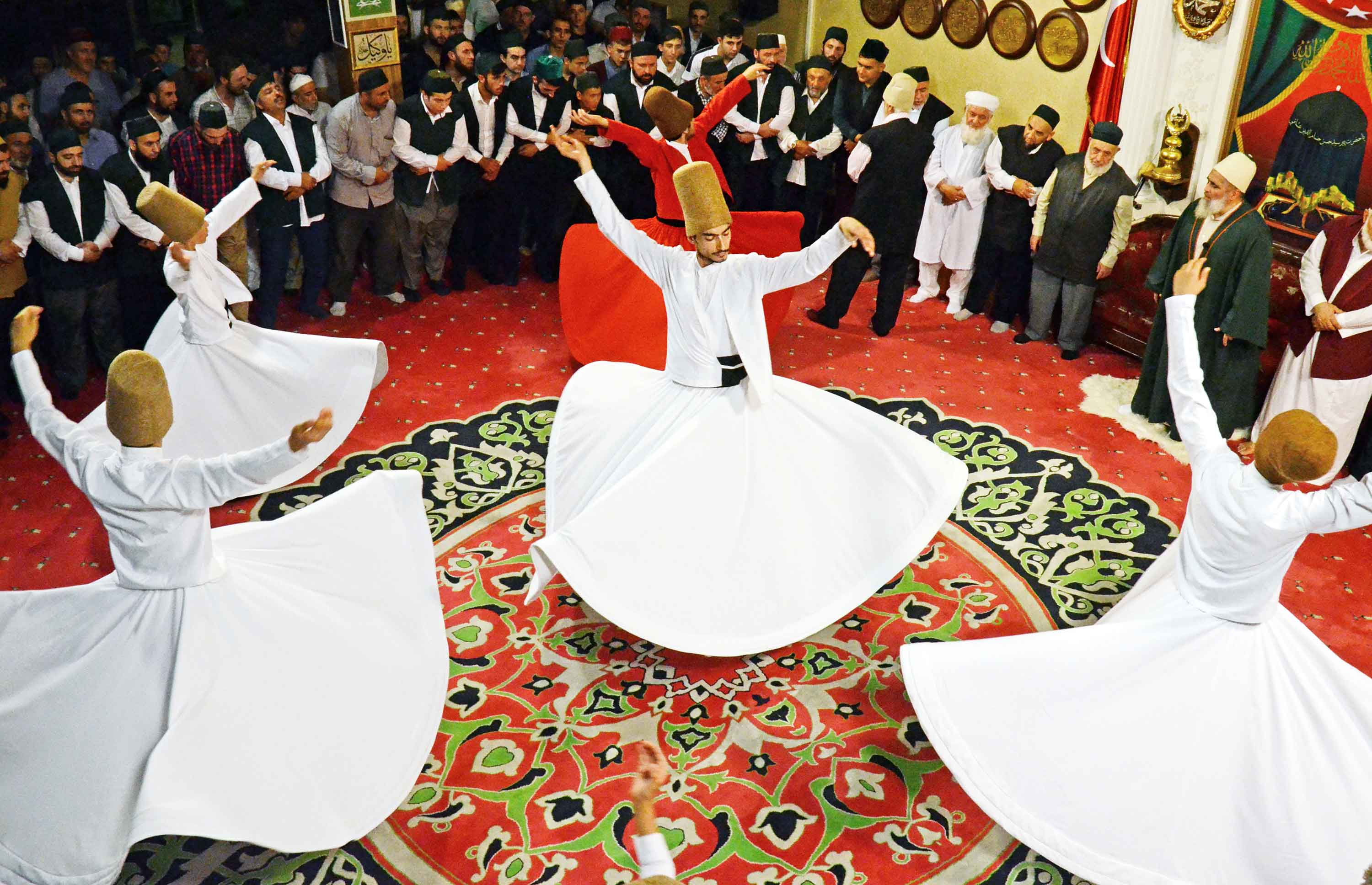The image captures a vivid and intricate Middle Eastern dance ceremony. At the center of a large, ornately patterned carpet predominantly colored in green, red, and cream, five men are performing a mesmerizing dance. Four of the men are dressed in traditional white costumes consisting of white jackets, thick black sashes around their waists, and long circular skirts that billow out as they spin with their arms raised in the air. One of the dancers stands out in a similar outfit but in a striking red hue. Each man wears a tall, yellowish-brown hat that adds to the traditional aesthetic.

The dancers are surrounded by several spectators, all of whom appear to be men with large beards, and many are wearing various hats or headdresses, indicating the cultural significance of the event. The background hints at a ceremonial or commemorative atmosphere with the presence of flags and numerous plaques adorning the space. The detailed carpet underfoot and the vibrant costumes create a colorful and dynamic scene that reflects the rich cultural heritage of the region.